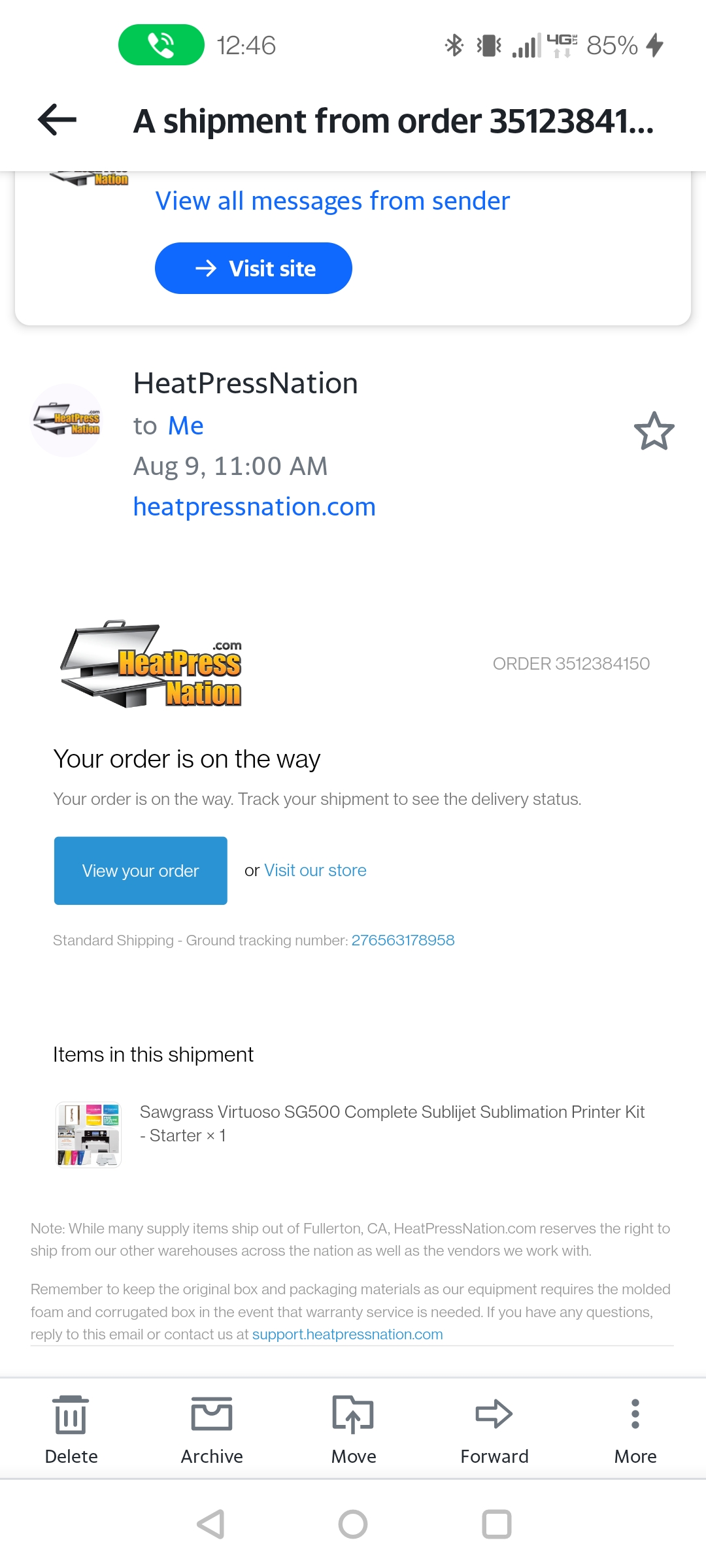Screenshot of an online shipment confirmation from Heat Press Nation. The screenshot features a white background and details for order number 35123841. The 85% battery icon with a thunder symbol is displayed, indicating the device's battery level. The current time shown is 12:46. 

The top section of the image includes a green oval icon with a white phone and a back arrow, indicating a previous navigation option. The text "shipment from order 35123841" is present. Below this, there's an option to "View all messages from sender" in blue text. A blue oval button with "Visit Site" in white text and an arrow pointing to the right is visible on the screen.

The email is from Heat Press Nation, received on August 9th at 11:00 a.m. A star icon precedes the text "heatpressnation.com." 

The main message reads "Your order is on the way," followed by the order number. There is a blue rectangle button with the text "Track Your Order" in white, and "Visit Our Store" in blue. It lists items in the shipment, including a Sawgrass product, along with additional item information.